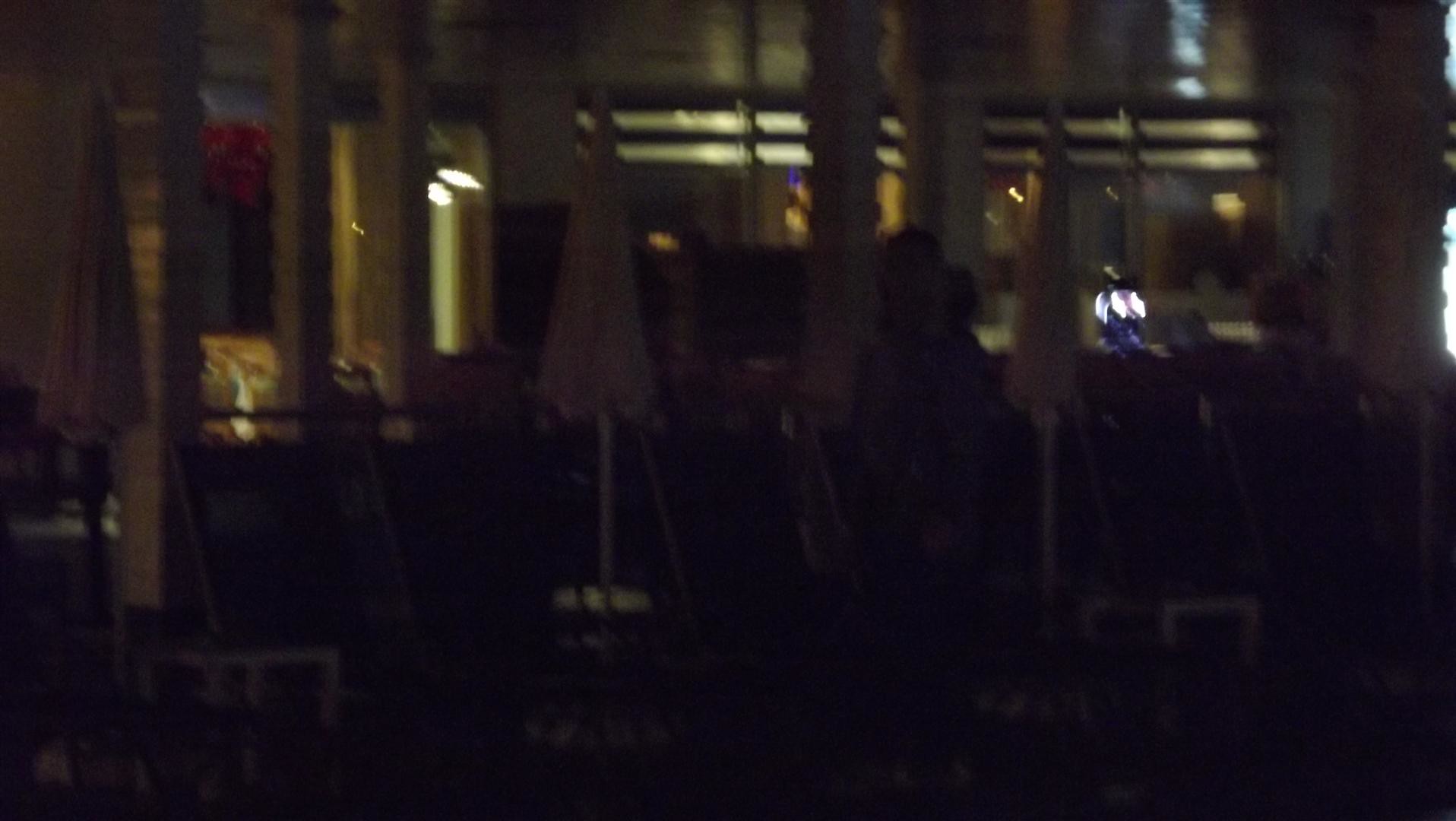A dimly lit outdoor patio of a closed restaurant at nighttime is captured in this image. The interior background of the restaurant is visible, though faintly illuminated by a few ceiling lights and a single light over a window, providing a soft, ambient glow. In the foreground, the patio furniture includes several tables, each accompanied by closed table umbrellas that appear to be a grayish-pink color. Although visibility is low due to the darkness, the silhouettes of approximately four umbrellas can be discerned. Slightly off-center to the right stands a figure, possibly a woman with shoulder-length blonde hair, dressed in a light-colored jacket. The scene is shrouded in shadows, rendering many details indistinct.